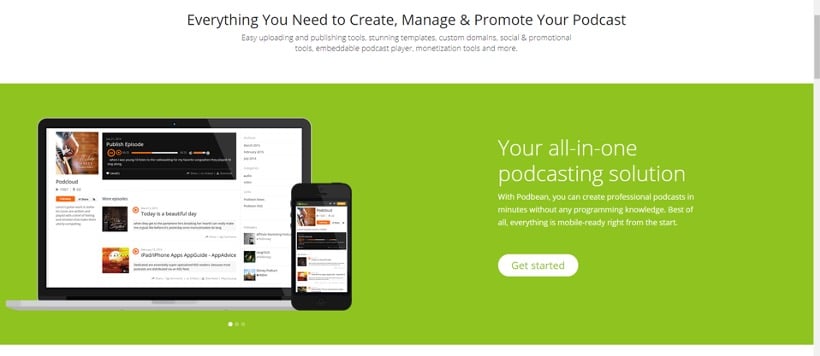This image is a detailed screenshot of a podcasting app interface. At the top, there is a prominent heading in dark, large font that reads: "Everything you need to create, manage, and promote your podcast." Below that, in smaller, non-bolded font, it lists key features: "Easy uploading and publishing tools, stunning templates, custom domains, social and promotional tools, embeddable podcast player, monetization tools, and more."

The upper third of the image features a white background. The lower section transitions into a green background, dominated by a large visual element on the left. This includes a laptop displaying a website, partially overlapped by a phone showing the same website, both indicative of a podcasting platform with clickable episodes.

To the right of these images, text reads: "You're all in one podcasting solution" in large letters, followed by smaller text: "With Podbean, you can create professional podcasts in minutes without any programming knowledge. Best of all, everything is mobile-ready right from the start." 

Beneath this text is a white oval button encapsulating the words "Get Started" in green, making it stand out against the green background. Most of the text throughout the image is white, aligning cohesively within the design.